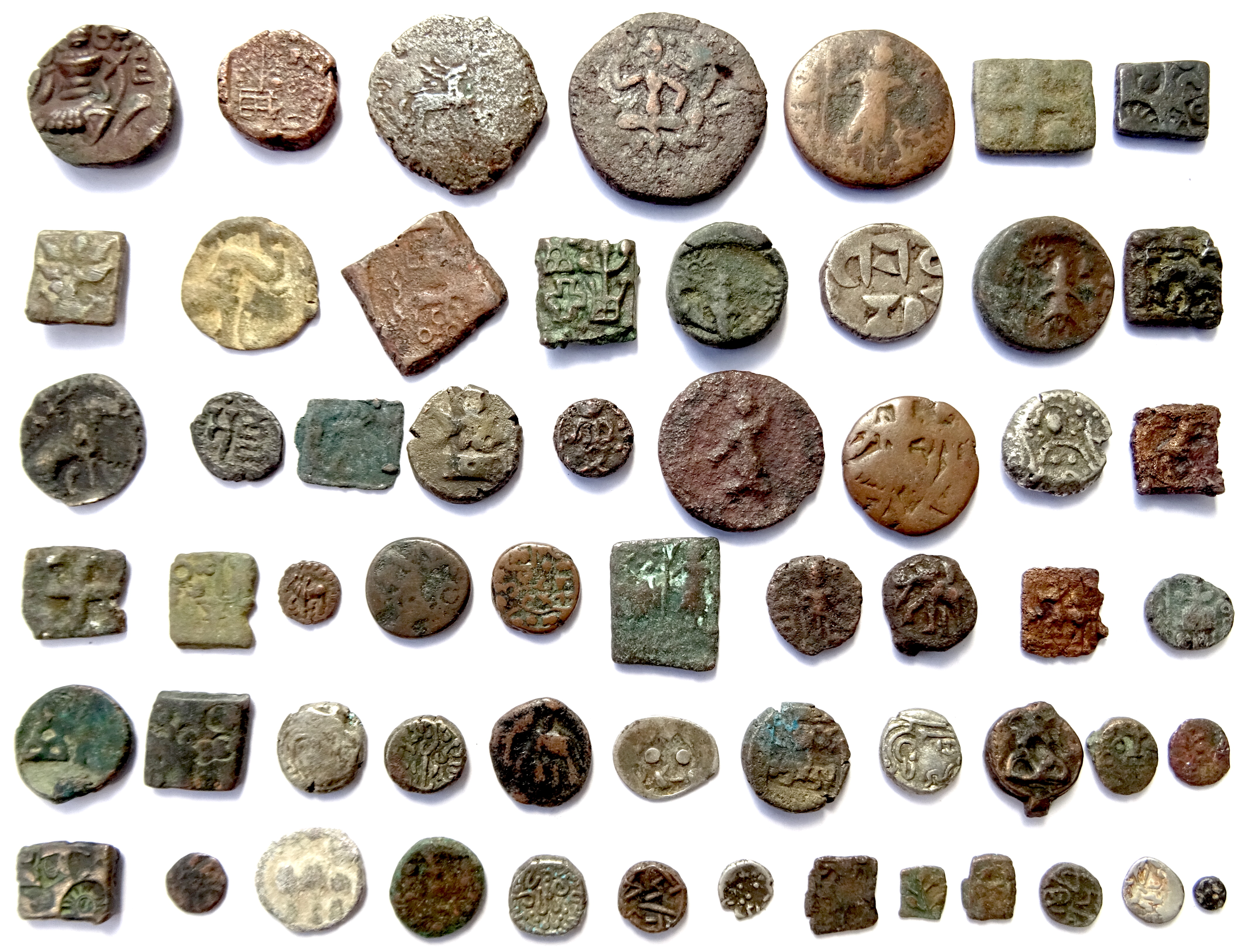This color photograph captures approximately 60 ancient coins, laid out in six rows against a white background. The coins vary in size, with the largest ones occupying the top row and progressively smaller ones in the descending rows. The coins also differ in shape, with most being circular while some are square, including a square coin turned at a 45-degree angle. They span a spectrum of colors including rust, brown, dark green, black, gray, silver, gold, and bronze, and show signs of aging such as pitting with rust and worn, smooth surfaces.

The intricacy of the coins is evident through various markings, which include pictures, faces, and etchings—though many carvings are now almost unreadable due to age. These coins, likely produced by hand rather than in a factory, possess an artifact-like quality, reminiscent of hieroglyphics. Their diversity in material, design, and origin showcases a rich history and illustrates the evolution of coinage across different areas and eras.